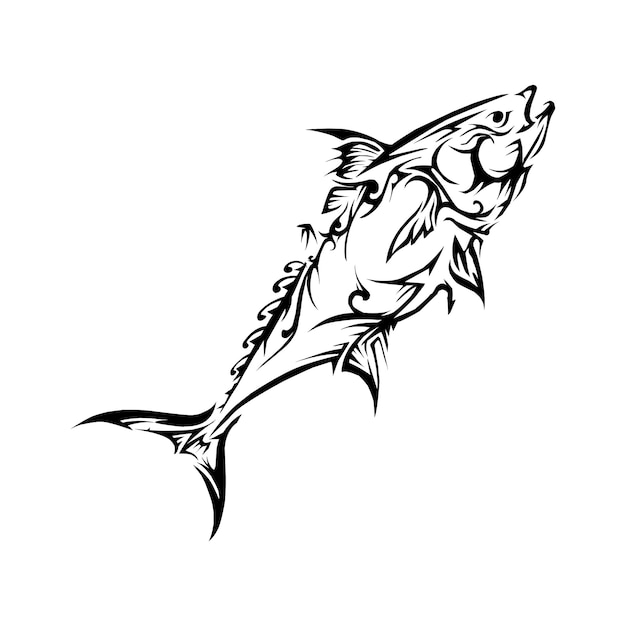The image portrays an abstract black-and-white line drawing of a stylized fish, rendered on a white background. The fish is depicted in a tribal tattoo-like design, characterized by bold black lines that outline and highlight its form. The fish is positioned diagonally, with its tail curving towards the bottom left corner and its head angling up to the top right. Although it has a finned tail, two fins on the back, and two fins on the front, the fish's texture and scales are suggested through intricate, curving, and geometric lines rather than lifelike details. Its mouth is open, creating the impression of gasping for air, and a single visible eye is wide open. The image's composition includes considerable white space, enhancing its artistic and abstract nature. No textual elements are present in the image.